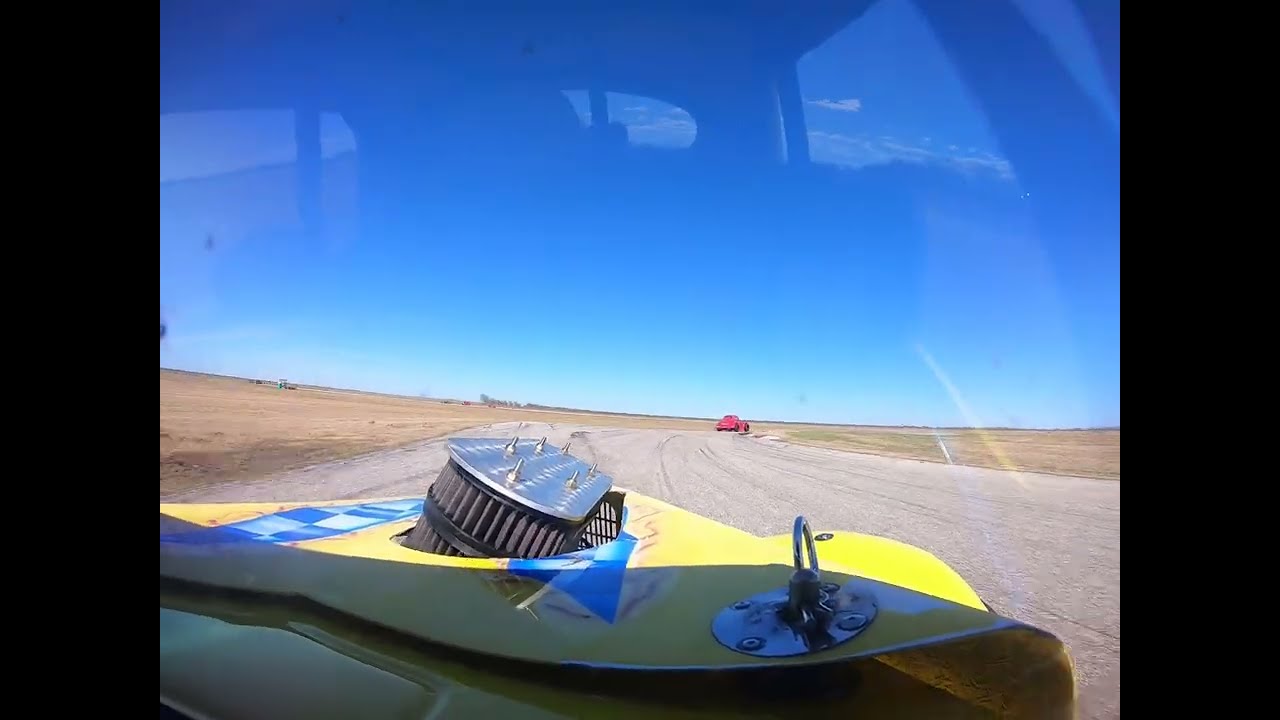From within the low-slung interior of a yellow and blue striped race car, a first-person perspective reveals the open road ahead. The car’s hood sports a protruding silver and black engine, featuring a prominent filter and a bolted metal circle on the right. The sleek dashboard inside is light gray, and reflections of the car’s interior dance on the windshield, merging with the clear, cloudless dark blue sky above. The asphalt road is bordered by patches of light brown dirt and light green grass. In the distance, a red pickup truck can be seen on the horizon, appearing small and far away against the rural backdrop.